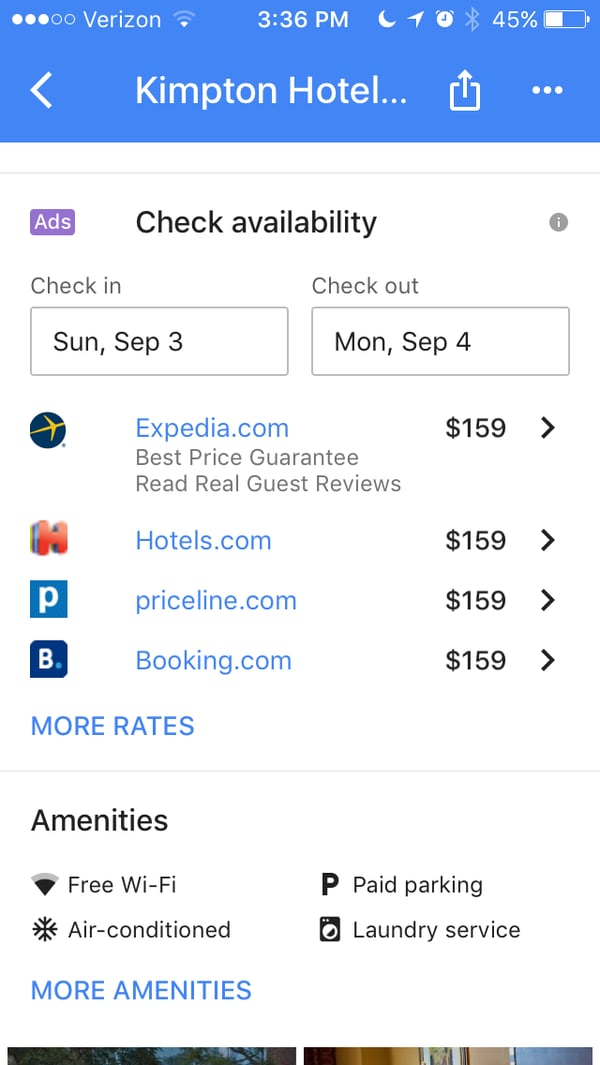At the very top of the image, there is a long blue bar. Within this bar, there are three filled white circles, followed by two open circles. To the right of these circles is the word "Verizon." In the center, the time is shown as 3:36 PM. Next to the time, icons of a moon and a clock or alarm are visible. Further to the right, "45%" is displayed alongside a battery icon that is halfway filled.

Below this section, on the left side, there is an airplane icon next to the text "Kempton Hotel," spelled K-I-M-P-T-O-N. Beneath this, the text reads "Check Availability," followed by "Check-in" and, inside a square, "Sunday, September 3rd." Below this is "Check-out," shown with the date "Monday, September 4th."

Further down, there is an airplane icon inside a blue circle, alongside the text "Expedia.com" and a price of "$159." Following this, the text "Hotels.com" appears with a price of "$159." Next is a "P" inside a blue square, followed by "Priceline.com" and the price "$159." A capital "B" inside a dark blue square is shown next to "Booking.com" with a price tag of "$159." The text continues with "More rates."

Below this, the text "Amenities" is listed, including "Free Wi-Fi," an image of a snowflake next to "Air Conditioned," "Paid Parking," and "Laundry Service." At the bottom of this section, in blue capital text, the words "More Amenities" are displayed.